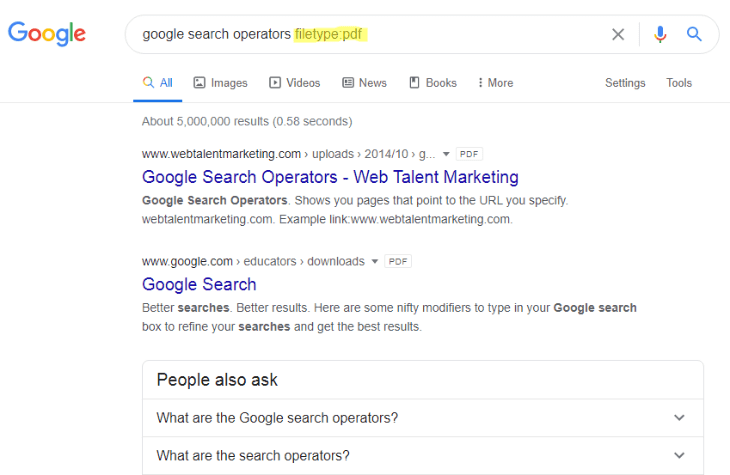A screenshot of a Google search results page appears, outlined within a square format. At the top of the page, the Google logo is prominently displayed in the upper left corner, adjacent to a search box containing the query "Google search operators file type: PDF." To the right of the search box, an "X" button, a microphone icon, and a magnifying glass icon for initiating the search are visible.

Directly below the search bar, a navigation menu offers the options: "All," "Images," "Videos," "News," "Books," and "More," with "All" highlighted in blue, distinguished by an underline, while the other options remain in dark gray text. On the far right of this menu, "Settings" and "Tools" options are accessible.

The search results indicate approximately 5 million results returned in 0.58 seconds. The primary result appears from webtalentmarketing.com, highlighting an article about Google search operators, with a brief description reading: "Google search operators show you pages that point to the URL you specify." Below this, another search result description suggests, "Better searches, better results. Here are some nifty modifiers to type in your Google search box to refine your searches and get the best results." This content introduces various techniques for improving Google search efficiency.